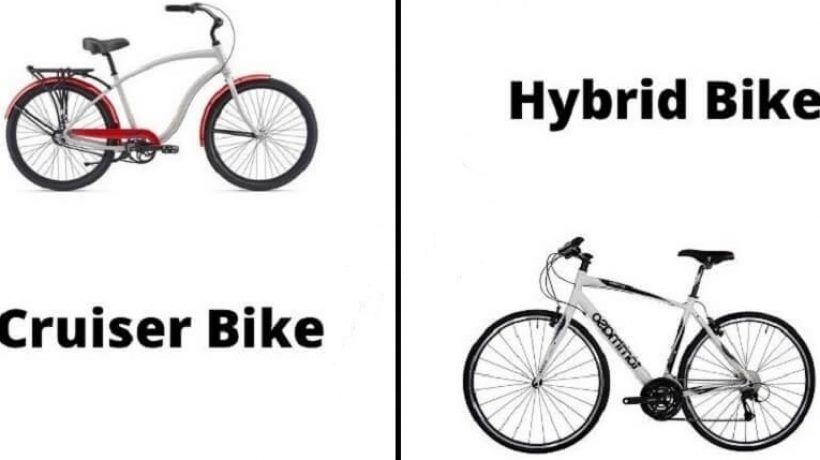The image depicts a comparative advertisement showcasing two distinct bicycle models positioned diagonally against a white background. In the upper left corner, a vintage-style cruiser bike, painted in red with white accents, faces towards the right. This bike features high, wide handlebars, a curved top bar, black tires and spokes with silver details, and a back fender supporting a small luggage rack. Black text beneath it labels it as a "cruiser bike."

In contrast, the lower right corner houses a sleek, black hybrid bike facing the left. This model is designed for more rugged, enduro-type use, featuring a minimalist frame without fenders, black brake lines, handlebars with integrated brakes and gears, and a streamlined appearance. The hybrid bike is characterized by its functional design, with black tires and a white top bar providing striking contrast. Above this bike, black text labels it as a "hybrid bike." A dividing line separates the two bikes, emphasizing their differences. The overall layout suggests this is likely part of a presentation or a website feature aimed at highlighting the unique attributes of each bike model.